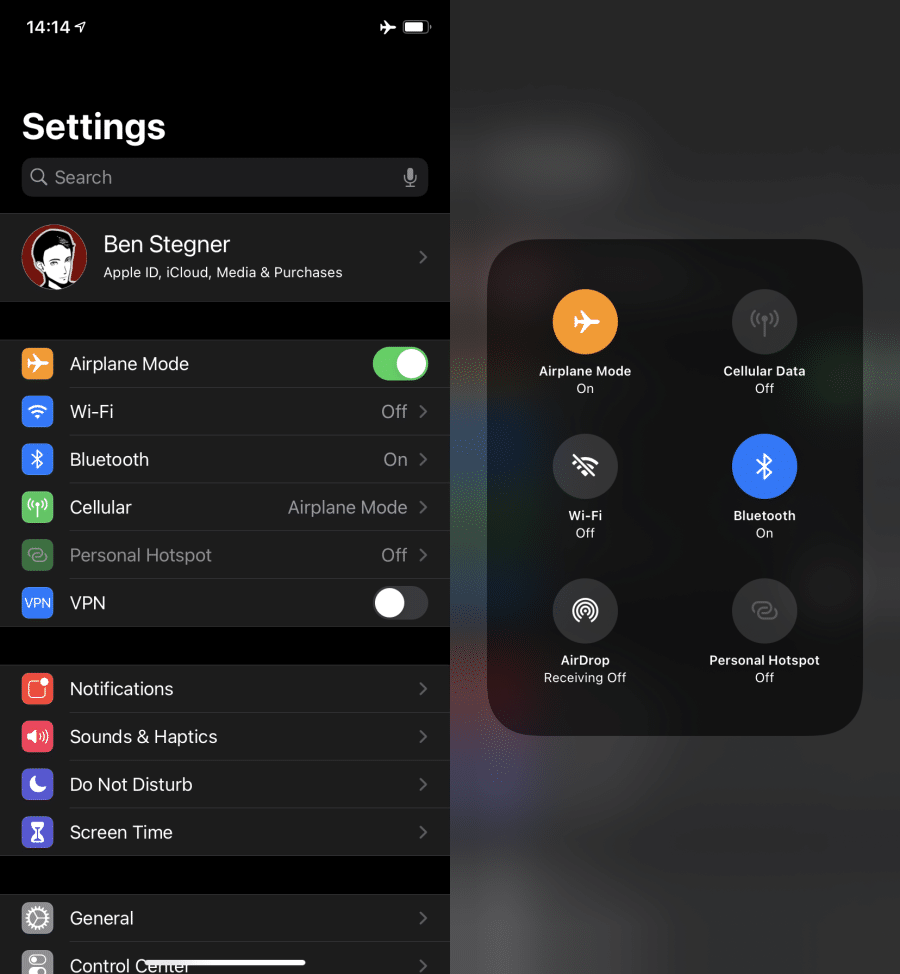This image is a screenshot of a mobile device's settings page, which is split into two columns with distinct background colors: a darker black for the left column and a lighter grayish tone for the right column. 

In the left column, at the top of the screen, the current time is displayed as 14:14. Adjacent to the time, icons for airplane mode and battery status are clearly visible. Below this, a sizable "Settings" header is accompanied by a search bar and an option for voice dictation. Continuing downward, the user's name, Ben Stegner, is displayed along with a profile picture, and there is an option to press the user's name for additional settings.

Further down, there are various settings options listed, including:
- Airplane Mode (currently toggled on)
- Wi-Fi
- Bluetooth
- Cellular
- Hotspot
- VPN
- Notifications
- Sounds
- Do Not Disturb
- Screen Time
- General Control Center

In the right column, quick setting icons for several features are arrayed, including:
- Airplane Mode (toggled on)
- Cellular Data
- Wi-Fi
- Bluetooth (toggled on)
- AirDrop
- Personal Hotspot

This detailed view provides a comprehensive look at the available settings and their current statuses on Ben's mobile device.